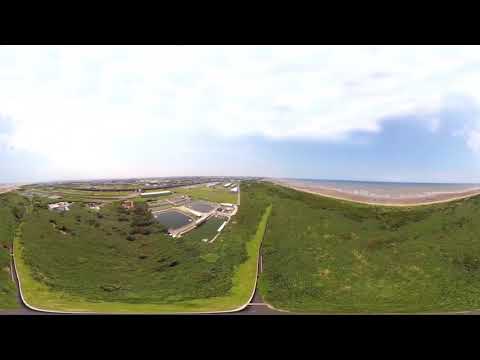The aerial photograph captures a landscape divided into two distinct sections. On the right side, a grassy hill slopes gently down to a distant, dark-colored ocean, bordered by a shoreline. On the left side, a large, circular pool—possibly part of a water treatment plant or sewer system—sits amidst patches of greenish grass that vary in shade, suggesting some areas may not be very healthy. Beyond this industrial structure, a faint glimpse of the city is visible on the horizon. A road runs down the center of the image, cutting between the grassy sections and leading up into the hill. The sky above is predominantly cloudy, with white, wispy clouds and the occasional patch of blue peeking through.